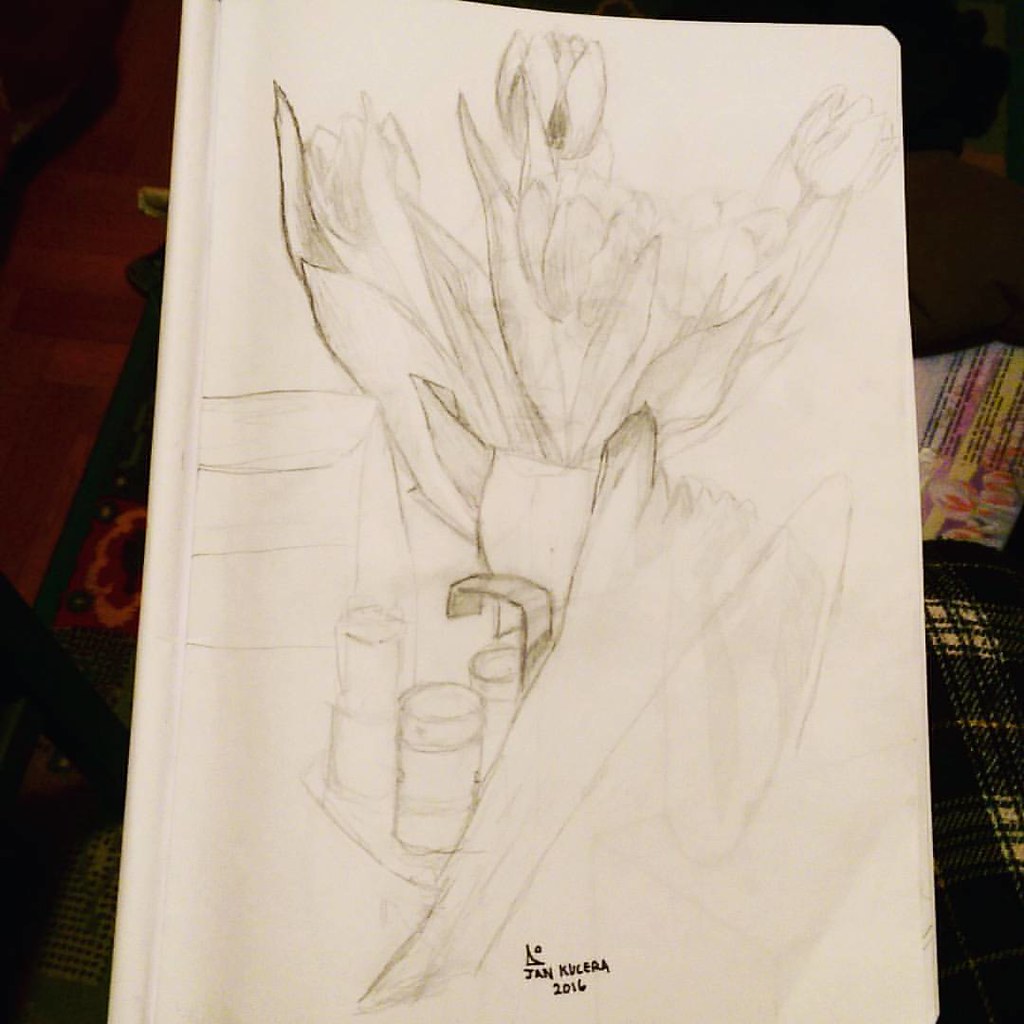This vertical pencil sketch, created by Jan Kuchera in 2016, depicts a vase of tulips placed beside a kitchen sink. The vase, situated centrally in the composition, holds three to four tulip blooms along with accompanying greenery. To the right of the vase, a few glasses, ringed with circular bands and likely positioned upside-down, are arranged next to an angular, flat-looking spigot. An assortment of indeterminate objects populates the surrounding area. The sketch is signed and dated by the artist at the lower center. The paper on which the drawing is made appears to be propped up against some object, possibly on a sofa, part of whose upholstery is visible on the right side of the image.